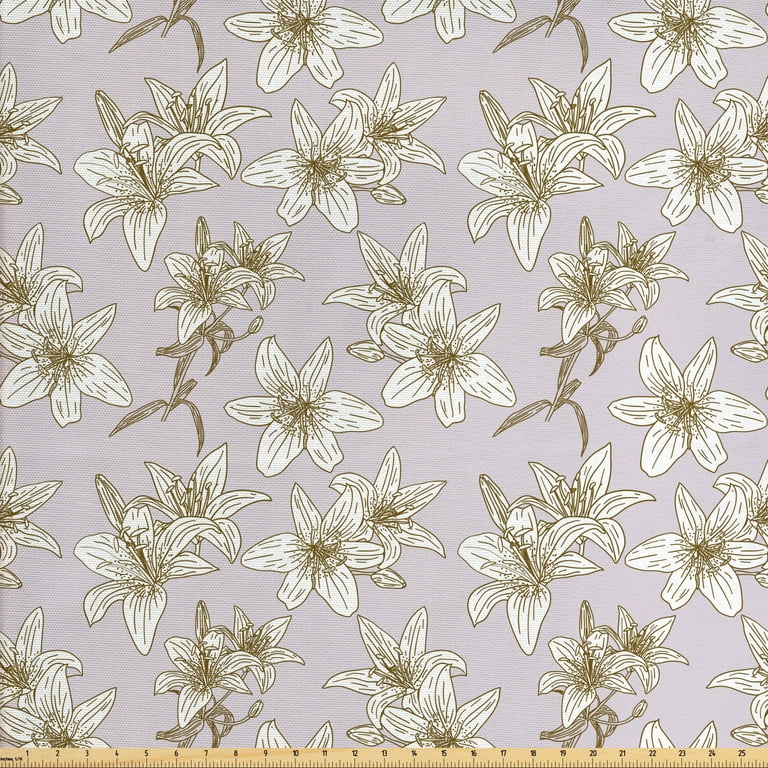This image features a possibly digitally rendered or stylized design reminiscent of fabric or wallpaper. The background is a light lavender, almost bluish-gray hue. Throughout the entire image, there are about 30 white flowers with six petals arranged in a star pattern. Each flower displays intricate details, including black lines that form the petals and burst outward from the center to depict the stamens and reproductive parts. The flowers are scattered randomly across the background rather than in rows. At the bottom of the image, a brown ruler spans from left to right, marked with measurements up to 25 centimeters.